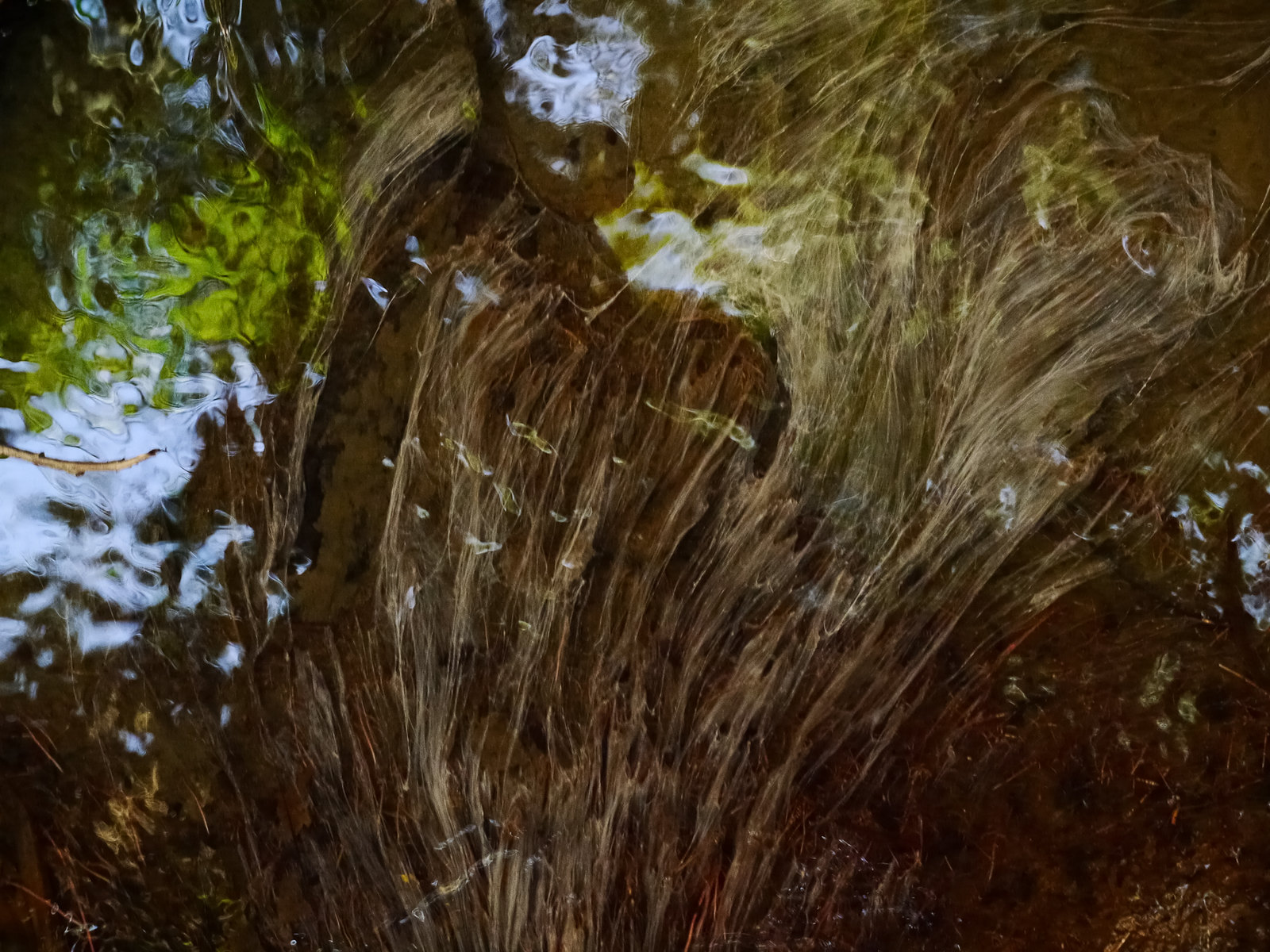The image depicts what appears to be a mesmerizing water scene, which could be either a photograph or a painting. The background showcases a dappled texture with green, light green mossy hues and scattered patches of water, creating an impression of ripples. The water surface might reflect the surroundings or demonstrate elements within it. The lower portion of the image transitions into dark, almost black and dark brownish-red shades, housing what seems to be vegetation. These vegetation elements include long, frond-like white leaves, possibly either submerged or reflected on the water's surface.

The scene projects an intricate play of reflections, with the upper region featuring reflective patches that hint at the sky's bluish tint, interspersed with reflections of light and potentially green trees. The overall color scheme integrates brown, blue, and green tones, with blue emerging prominently on the right side, the middle, and the top left corner. A patch of green can be noticed near the upper left corner. Additionally, the presence of two brown eye-like shapes near the upper right, alongside a silhouette resembling an owl perched on a tree, adds an element of intrigue and whimsy, enhancing the image’s depth and complexity.